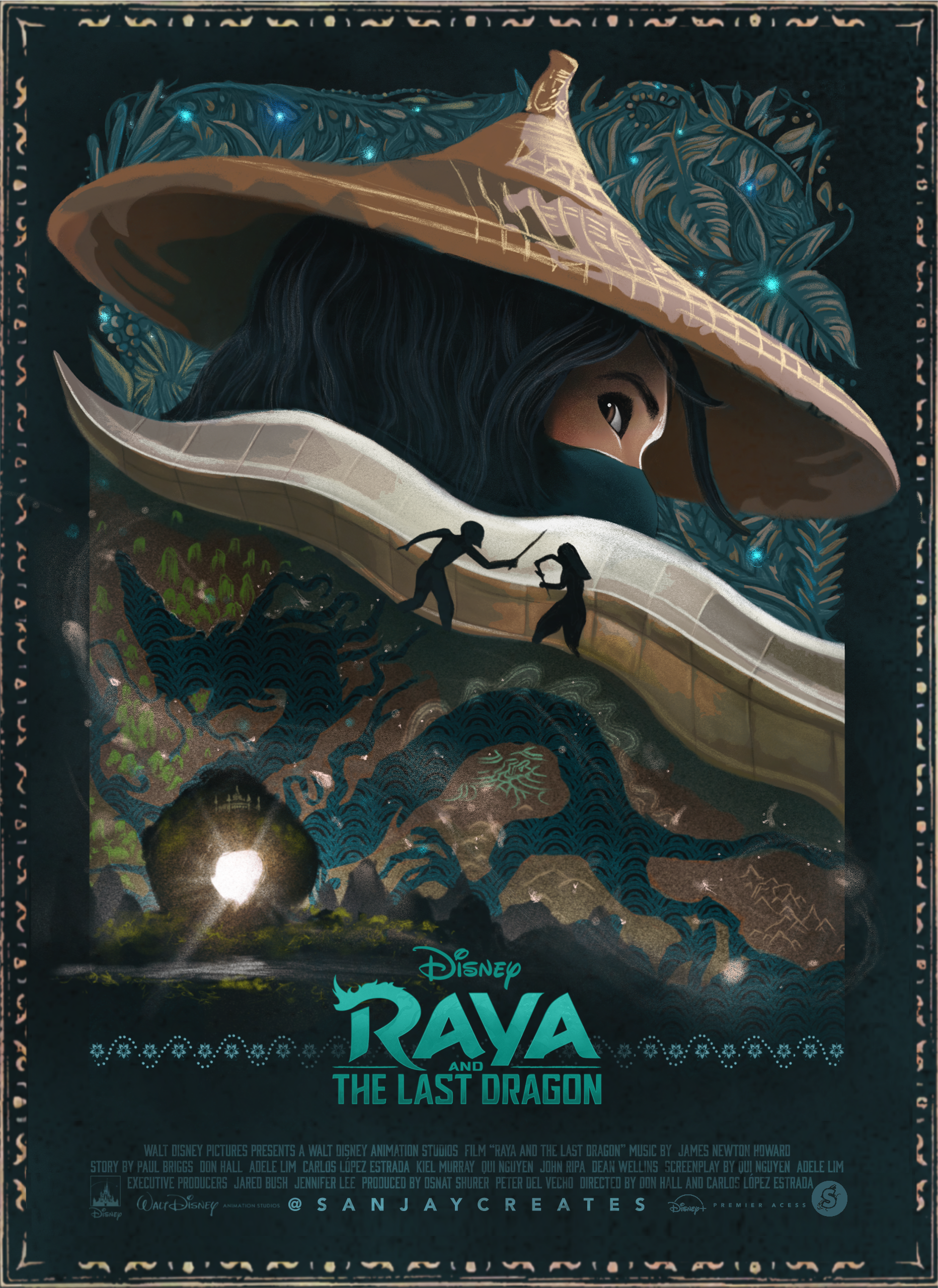This is a detailed movie poster for Disney's "Raya and the Last Dragon," framed with an intricate golden border featuring squiggly patterns. The dominant color palette includes dark and light blues, greens, browns, with shiny little lights adding vibrancy. At the center of the poster is the main character, Raya—a girl with thick, curly black hair. She is wearing a traditional Asian sun hat made of brown straw and partially concealing her face with a green mask. Her visible eye and eyebrow are brown, looking towards the right.

In the background, swirls of leaves in blue hues add a mystical touch, intertwined with shiny lights. The landscape is subtly illustrated, showing nature and a river that forms a dragon-like shape. The shadowy outline of a dragon runs across the image, serpentine in form with long claws, adding a sense of mystery.

Near the center, an artistic depiction shows two figures fighting, visible in the blade of a dagger or sword-like weapon. One figure wields a sword while the other has outstretched arms, grasping a smaller device.

The bottom of the poster contains essential details about the film including the title "Raya and the Last Dragon" in blue text, and credits mentioning Walt Disney Pictures, Walt Disney Animation Studios, and music by James Newton Howard. The overall composition is rich in detail and artistry, encapsulating the adventurous and magical essence of the film.